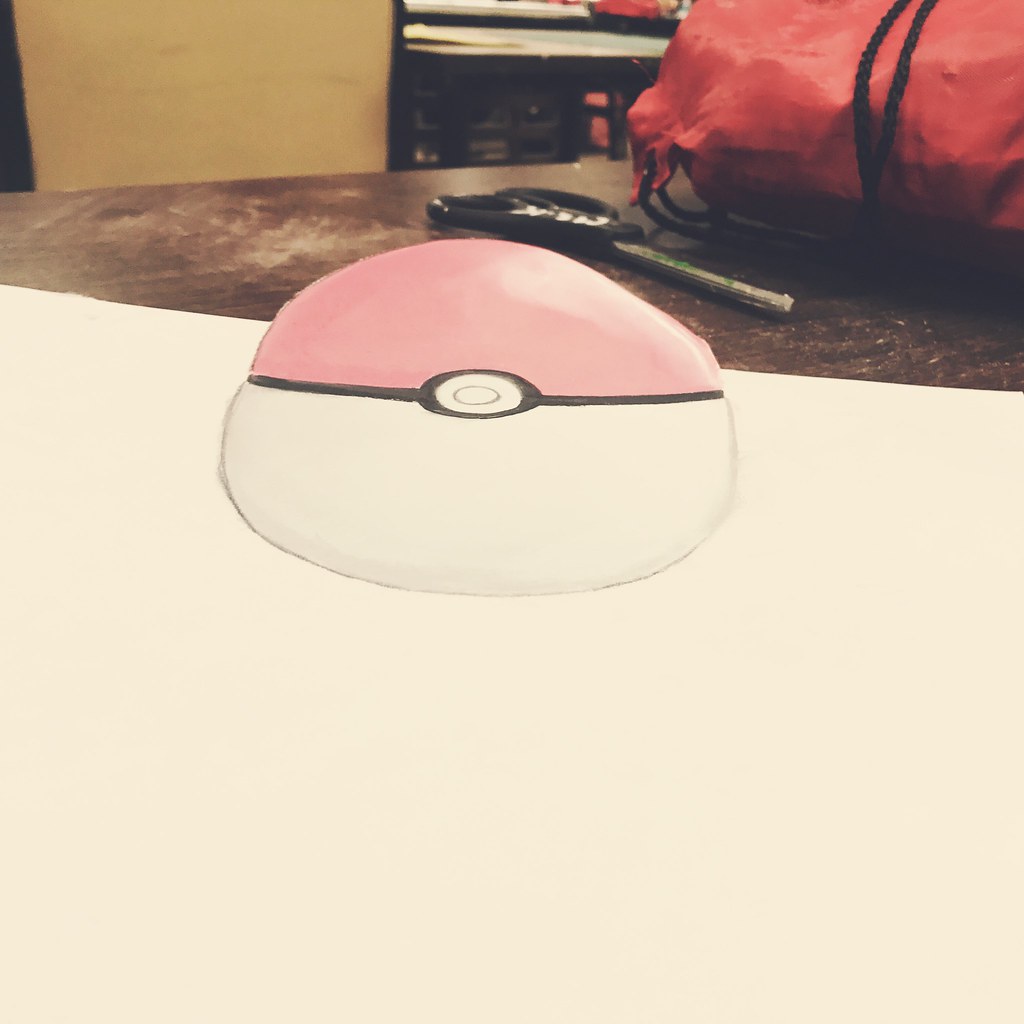This photograph captures a classroom setting where a handcrafted Pokéball art project is prominently featured. The Pokéball, distinguished by its iconic white and red halves separated by a black band, occupies the center of the image. It lays partially on a large sheet of white paper or a mat, spilling over onto a wooden desk. A pair of scissors, likely used to cut out the Pokéball, rests behind the artwork, evidencing the effort put into its creation despite slight imperfections in its circular shape. The background reveals a typical classroom ambiance, with red drawstring backpacks on the table, scattered chairs, and additional desks, indicating an environment bustling with student activity and creative endeavors.